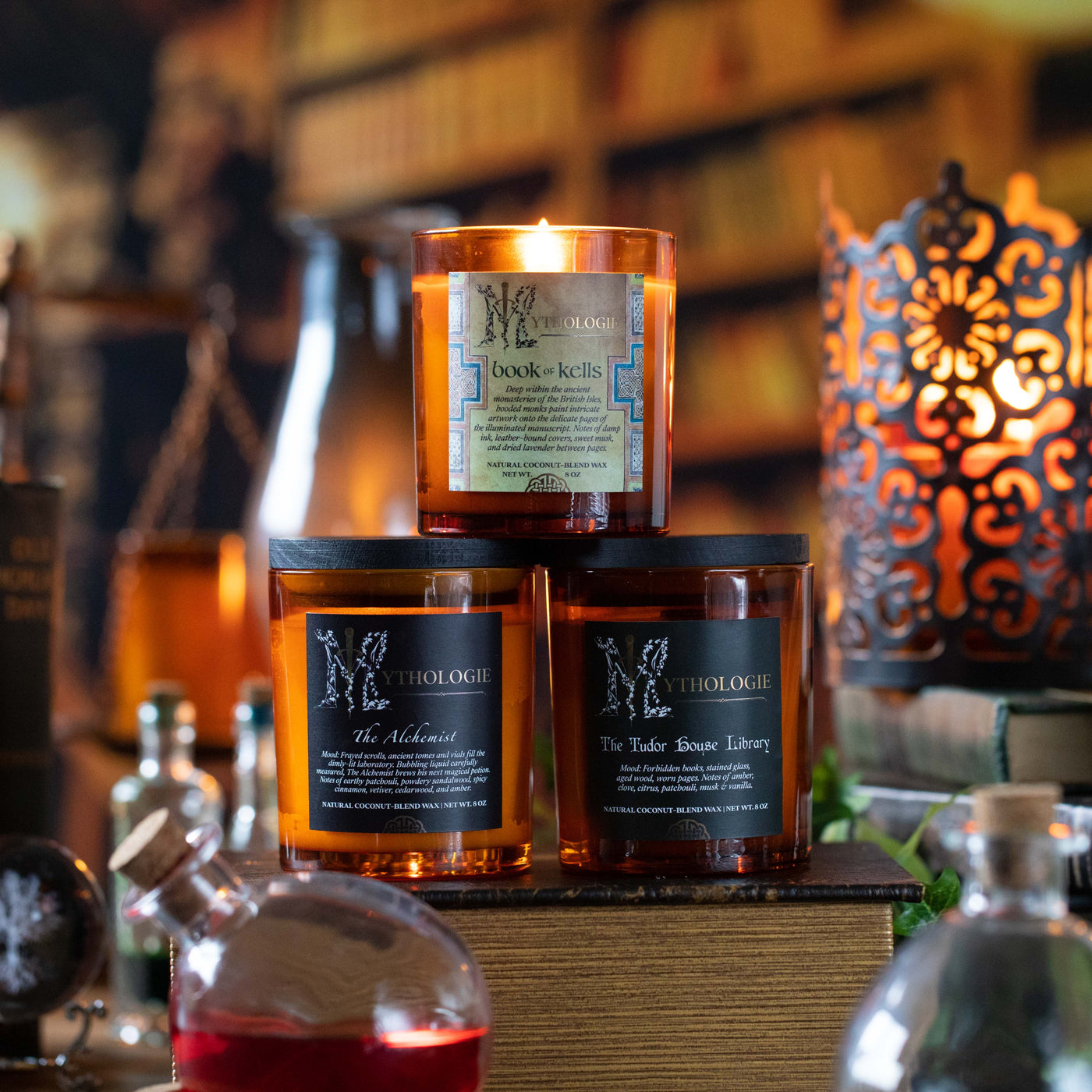In this full-color, square photograph taken indoors, natural and artificial light illuminates an eclectic collection of items, predominantly in hues of brown and red. Central to the image are three round, squat glass jars arranged pyramid-style atop a brown book with gold-edged pages. The book itself has a rich, brown leather cover. The two jars at the bottom have flat black lids and labels reading "The Alchemist" and "The Tudor House Library," both part of a candle collection labeled "Mythologie," spelled with an I-E. The jar at the top has a lit candle with a lighter label that says "Book of Kells," and describes intricate artwork and scents inspired by ancient British monasteries, with notes of ink, musk, and lavender. Nearby, at the upper right, is another lit candle inside a decorative metal frame, standing on a book. The lower corners of the image feature two glass bottles with cork lids, and additional bottles can be seen in the blurred brownish background, completing the atmospheric scene.